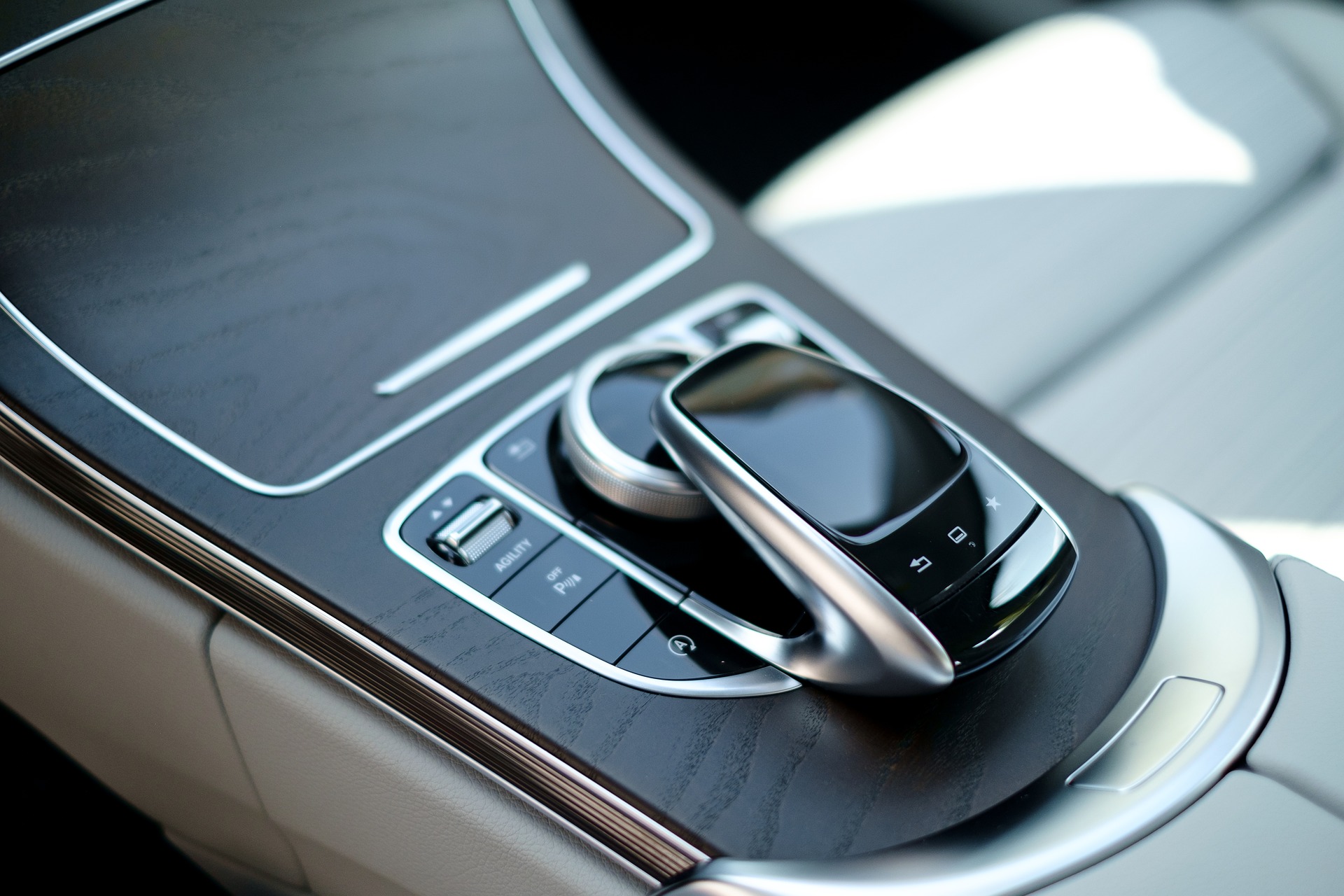This image captures the interior of a modern vehicle, specifically the center console area between the driver and passenger seats. The console features a prominent rectangular control display, resembling a smartphone, with a black screen occupying the upper half. This display includes functional buttons for navigation with icons for 'go back,' 'screen,' and 'start,' bordered by a distinctive black ring. Surrounding this display are additional buttons: on the left side, labeled 'Agility,' an 'off' button with a 'P' symbol, and a warning sign with a circular arrow. The right side features more buttons, although their exact functions are obscured. Below this setup is a circular knob likely used for adjusting settings, suggesting an advanced and possibly integrated infotainment or vehicle system. Above the main control area are small storage compartments, suitable for holding small items like keys or gloves. This high-tech console is accented by the luxurious touch of white leather seating, indicating a sleek and sophisticated vehicle design.